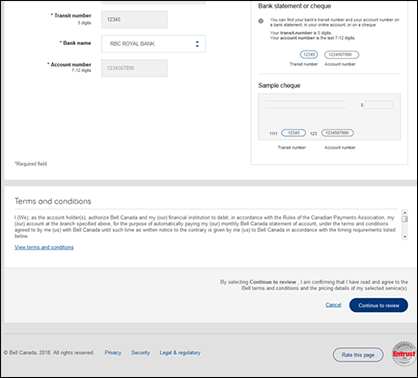The image depicts a small box filled with various pieces of text and information structured in multiple sections. Starting at the top left corner, there is a tiny black text labeled "Transit Number," accompanied by a box filled with the default numbers “12345.” Below that, the text reads "Bank Name" with "ABC Royal Bank" mentioned next to it. Further down, there is an "Account Number" field displaying the default numbers "1234567890."

To the right of these details, there is a header titled "Bank Statement or Check" followed by a small paragraph of information. Below this section, the text "Sample Check" is displayed. On the same top level, there is a set of "Terms and Conditions" described in a small black paragraph. Underneath, a blue, clickable link labeled "View Terms and Conditions" is provided.

Moving on to the bottom segment of the box, there is a small black text at the bottom right stating, "By selecting continue to review, I'm confirming that I have read and agreed to the terms and conditions and the pricing details of my selected service." Following this, options to "Continue to Review" or cancel are presented. At the very bottom, there is a final section displaying links for "Bell Canada," "Privacy," "Security," "Legal," and an option to "Rate This Page."